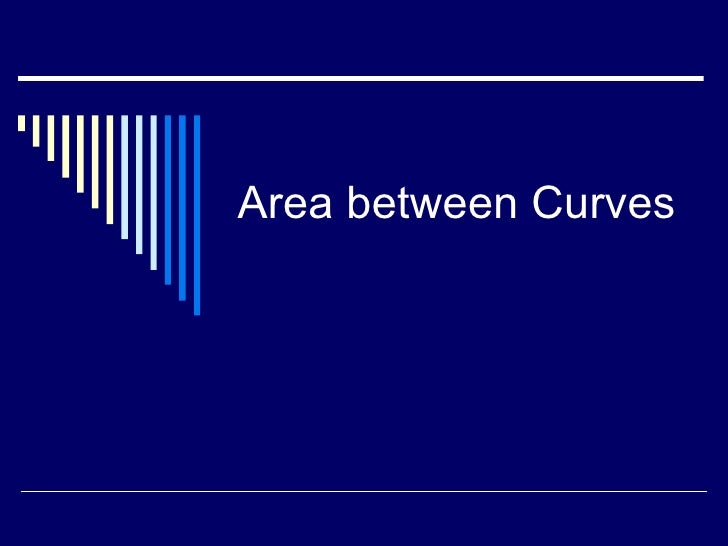The image is a rectangular PowerPoint presentation slide with a solid royal blue background. At the top of the slide, there is a near-horizontal white line running across most of the width, stopping just short of both edges. Below this white line, on the left side, there is a sequence of vertical lines that resemble a waterfall or an inverted barcode. These lines start with shorter white bars on the far left, progressively getting longer, transitioning through light blue, and culminating in longer bright blue bars, with the tallest reaching the center of the slide. Centered horizontally in the middle of the slide is the text "Area Between Curves" in a white sans-serif font, with 'Area' and 'Curves' capitalized while 'between' remains in lowercase. At the bottom of the slide, another very thin horizontal white line runs close to the slide's width, again stopping just short of both edges. There are no other texts or graphics on the slide.